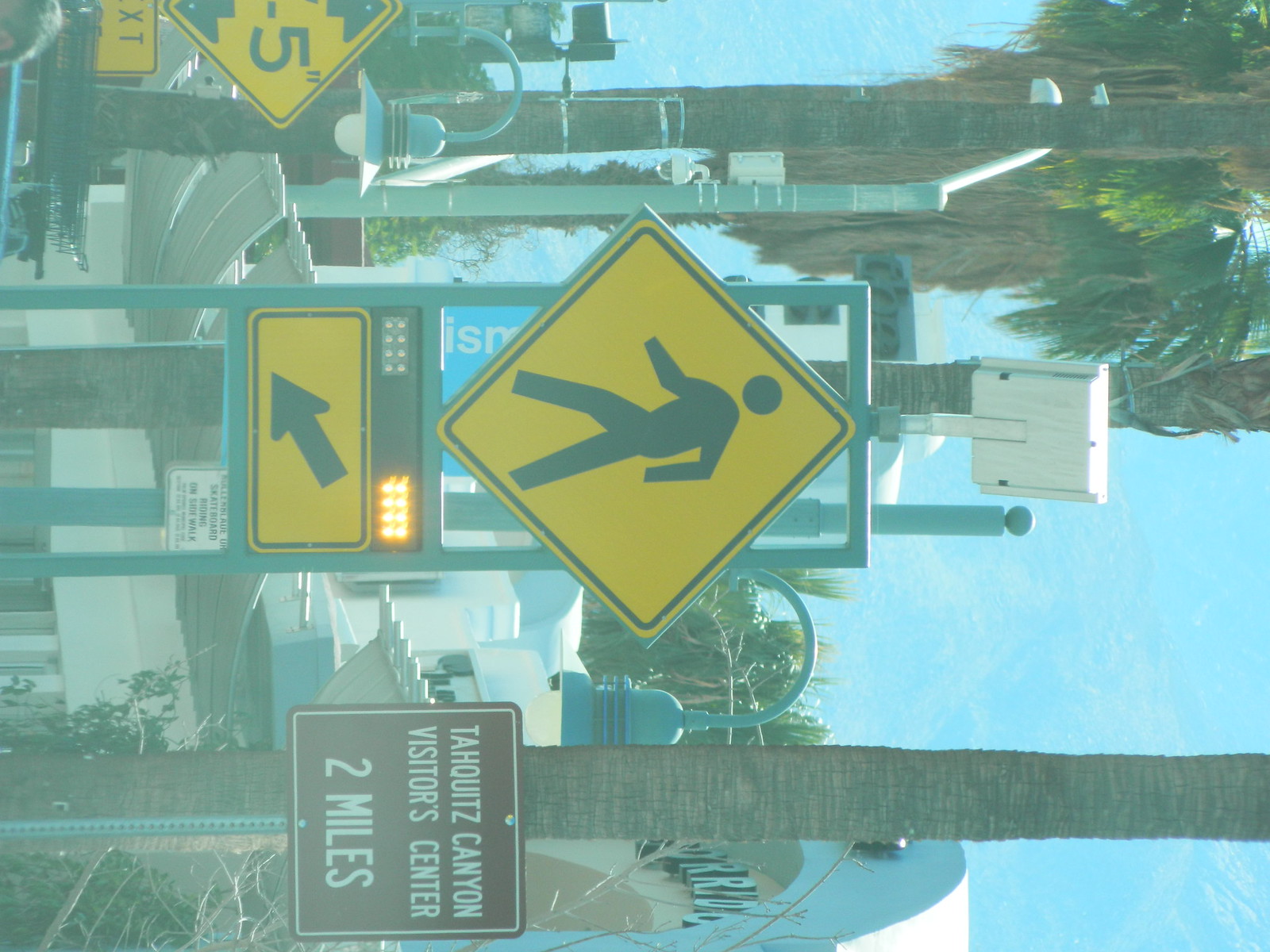This is a color photograph that appears quite faded and muted, possibly due to a filter or underexposure. The image is rotated 90 degrees to the right, requiring viewers to turn their heads to see it upright. Central to the composition is a yellow diamond sign with a black border, depicting a pedestrian symbol. Below this sign, there is a smaller rectangular sign with an arrow pointing left and slightly downward. To the upper left of these signs is a blown-out fluorescent display in an orange-yellow hue, rendering it unreadable. To the right, there's a brown square sign with white text that reads, "Tahquitz Canyon Visitor Center, 2 miles," positioned in front of a large tree trunk. In the background and to the right, there are faded blue skies and some buildings, one resembling a curved aircraft hangar. Palm trees and their leaves appear to the upper left, further suggesting a Californian setting, likely Palm Springs given the reference to Tahquitz Canyon. Additionally, the lower left corner shows the edge of another diamond sign with the number "5" under a curved light. The scene is busy with various streetlights, lampposts, and signs, capturing a bustling street intersection without any visible people.